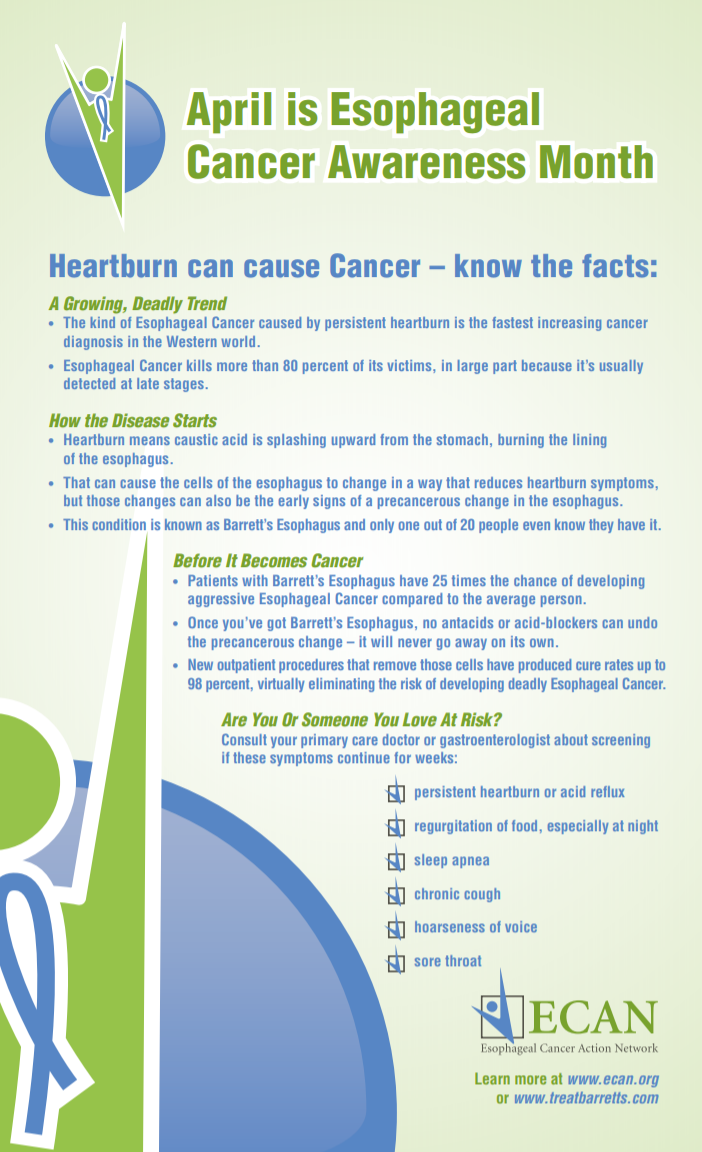The image is an educational poster with a pale green background featuring information about esophageal cancer awareness. At the top, in slightly darker green text across two lines, it announces "April is Esophageal Cancer Awareness Month." In the upper left corner, there's a blue circle with a green, V-shaped logo resembling a person with a circular head holding their arms up, accompanied by a blue ribbon symbolizing cancer awareness. Below the main heading, a key message states, "Heartburn can cause cancer. Know the facts." This is followed by an overview highlighting that esophageal cancer, particularly caused by persistent heartburn, is the fastest increasing cancer diagnosis in the Western world and has a high mortality rate due to late detection.

Further details include descriptions of how heartburn, caused by caustic stomach acid splashing up into the esophagus, can lead to cell changes that might become pre-cancerous, a condition known as Barrett's esophagus. Only one in twenty people with this condition are aware they have it. The poster features multiple green headings and several paragraphs explaining the disease, its symptoms, and the importance of early detection.

Additionally, there are bullet points in the lower right corner listing symptoms such as heartburn, regurgitation, sleep apnea, chronic cough, hoarseness, and sore throat, urging people to consult their primary doctors if they experience these signs. At the bottom, the green letters "ECAN" appear alongside the logo, and in the lower left corner, part of the logo is shown again, showing a blue circle with the green figure and blue ribbon. Further information can be accessed on the website: www.ecan.org.